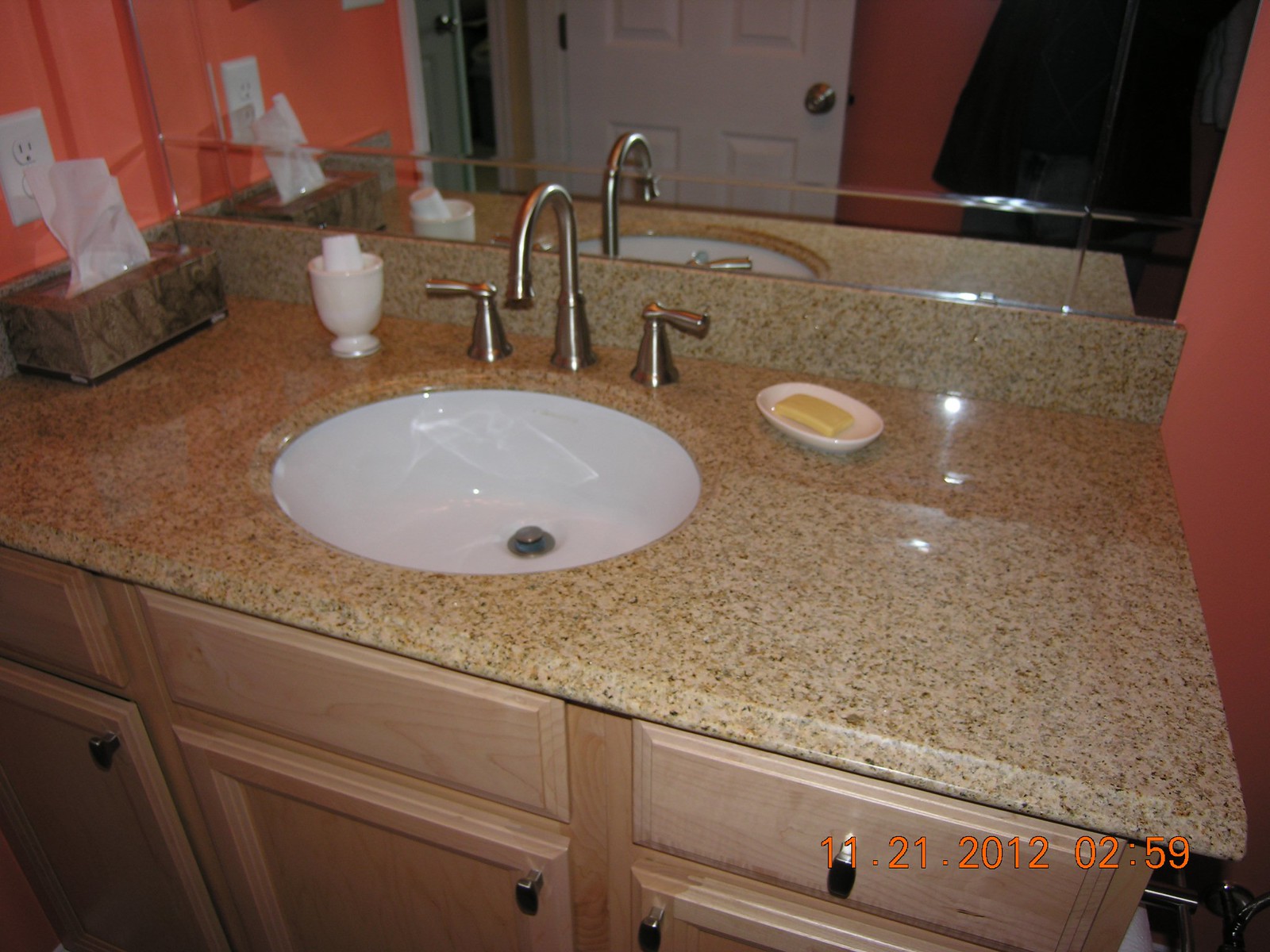This photograph features a well-lit bathroom sink area with a coral pink room in the background. The reflective mirror captures the photographer from their mid-chest to just above their thighs. The sink countertop is a luxurious beige and gold granite marble. In the back left corner near an electric plug-in, a Kleenex tissue box adorned with its signature brown swirls adds a touch of practicality. To the left of the sink, a white ceramic cup holds what appears to be a white bar of soap. The sink itself features a modern chrome faucet and a classic white bowl design. To the right of the sink, a white dish holds a yellow bar of soap. The bathroom vanity is made of light wash pine wood, lending a fresh and airy feel to the space. A small portion of the tissue paper holder is visible in the bottom right corner of the image. The bottom of the photo is timestamped with the date "11-21-2012" and the time "2:59," preserving the moment in time.